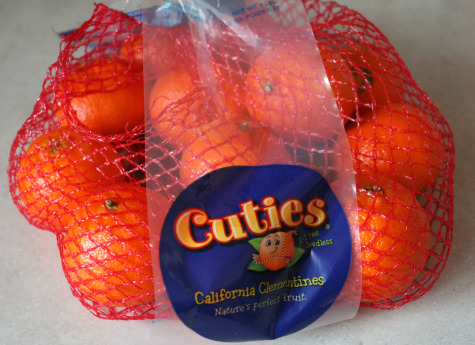The image features a bag of mandarin oranges branded as "Cuties." These California clementines are packaged in a red netting that fully encloses the oranges. The oranges, smaller than regular oranges, are similar in taste and appearance to mandarin oranges. The packaging also includes a clear plastic label wrapping around the bag. On this label, there's a navy circle housing the brand name "Cuties" in orange lettering. The logo on the label depicts a clementine with two eyes and a couple of leaves, alongside the text "California Clementines." There are additional, unreadable text elements on the label. The bag rests on a surface with a neutral cream or beige background.